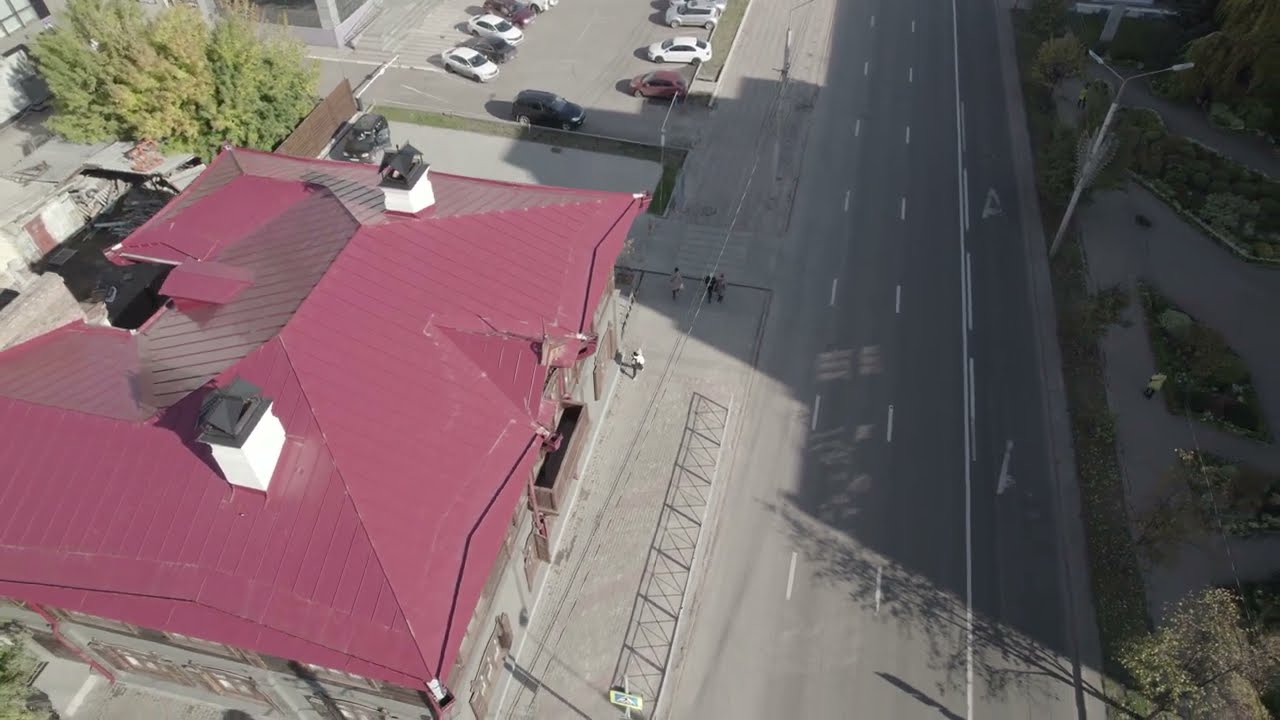This overhead image, possibly taken from a tall building, a drone, or a low-flying helicopter, prominently features a large building with a burgundy or purple metal roof situated at the lower left corner. The roof is distinguished by two white smokestacks with gray tops and has a slight peak in the middle. Just beyond this building, towards the top left, there is a small cluster of trees. Above these trees, in the upper left-hand corner, there is a parking lot filled with several cars, including white, red, silver, and black vehicles, with a notable black SUV visible.

To the right of the building, the image shows a three-lane roadway, which includes a bike lane with a solid white line and directional arrows. The road features scattered white stripes and a solid center line but has no visible traffic. Further right, there is an area that appears to be a park or walkway, with cement pathways winding through patches of green, and streetlights with lights extending left and right. The detailed landscape and the varied urban elements provide a vibrant view of this location from above.